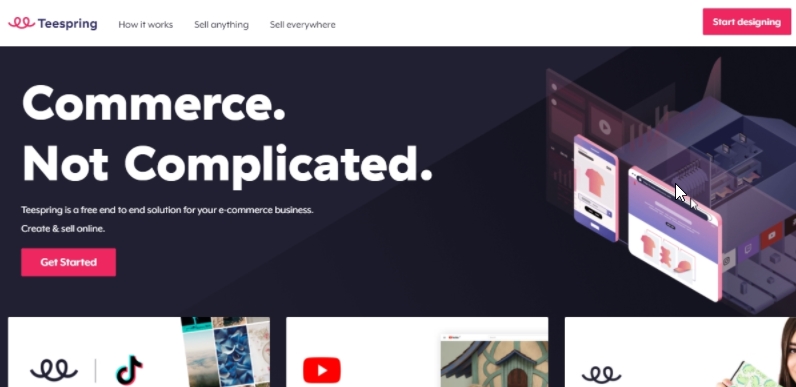The web page's header prominently displays the name "Teespring" in bold letters. To the right, there are three navigational links: “How It Works,” “Sell Anything,” and “Sell Everywhere.” On the far right, a vibrant pink button with white text invites users to "Start Designing."

The main body of the page features an engaging photo illustration of the product and services, set against a dark purple background. The central tagline, “Commerce, Not Complicated,” stands out in white font, followed by the subtext, “Teespring is a free end-to-end solution for your e-commerce business. Create and sell online.” Directly below, another prominent pink button, also with white text, urges visitors to "Get Started."

At the very bottom of the screen, there are three partially visible images that hint at social media integration and showcase various products and services offered by the platform. The cut-off photos suggest a visually rich representation of Teespring's offerings and capabilities.